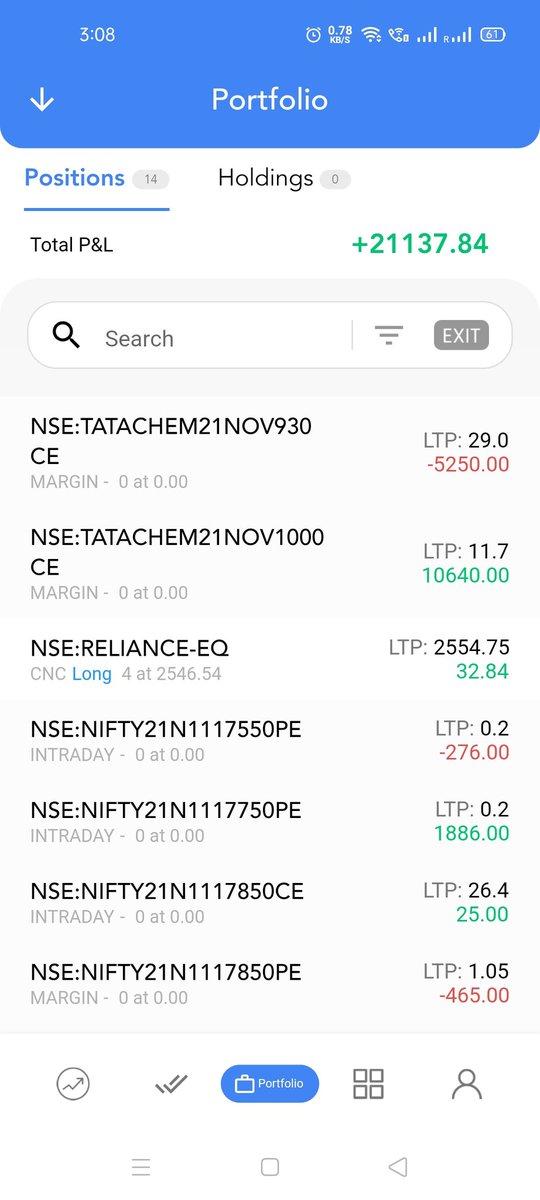A detailed screenshot of a smartphone displaying a financial portfolio application. At the top, a blue notification bar shows the time as 3:08, along with icons for the clock, Wi-Fi signal strength, cellular signal bars, and battery life. Below, a white downward-pointing arrow and the word "Portfolio" are prominently displayed. Immediately under this, the section labeled "Positions" indicates 14 total holdings and 0 current positions, highlighted with a blue underline.

Further down, a summary labeled "Total P&L" is shown, with a profit of +211.37 or 84%. Adjacent to this is a search bar with an "Exit" option on the right side. The main content consists of detailed listings for seven different stock tickers, each accompanied by "Margin 0 at 0.00," reflecting no margin used. On the right hand of each ticker, "LTP" (Last Traded Price) is followed by numbers in black, red, or green, denoting current stock prices or percentage changes.

At the bottom, a series of icons includes a crooked arrow, a circle, two check marks, a blue oval button labeled "Portfolio," a small user icon, and four small boxes arranged into a larger square, likely for navigation purposes.